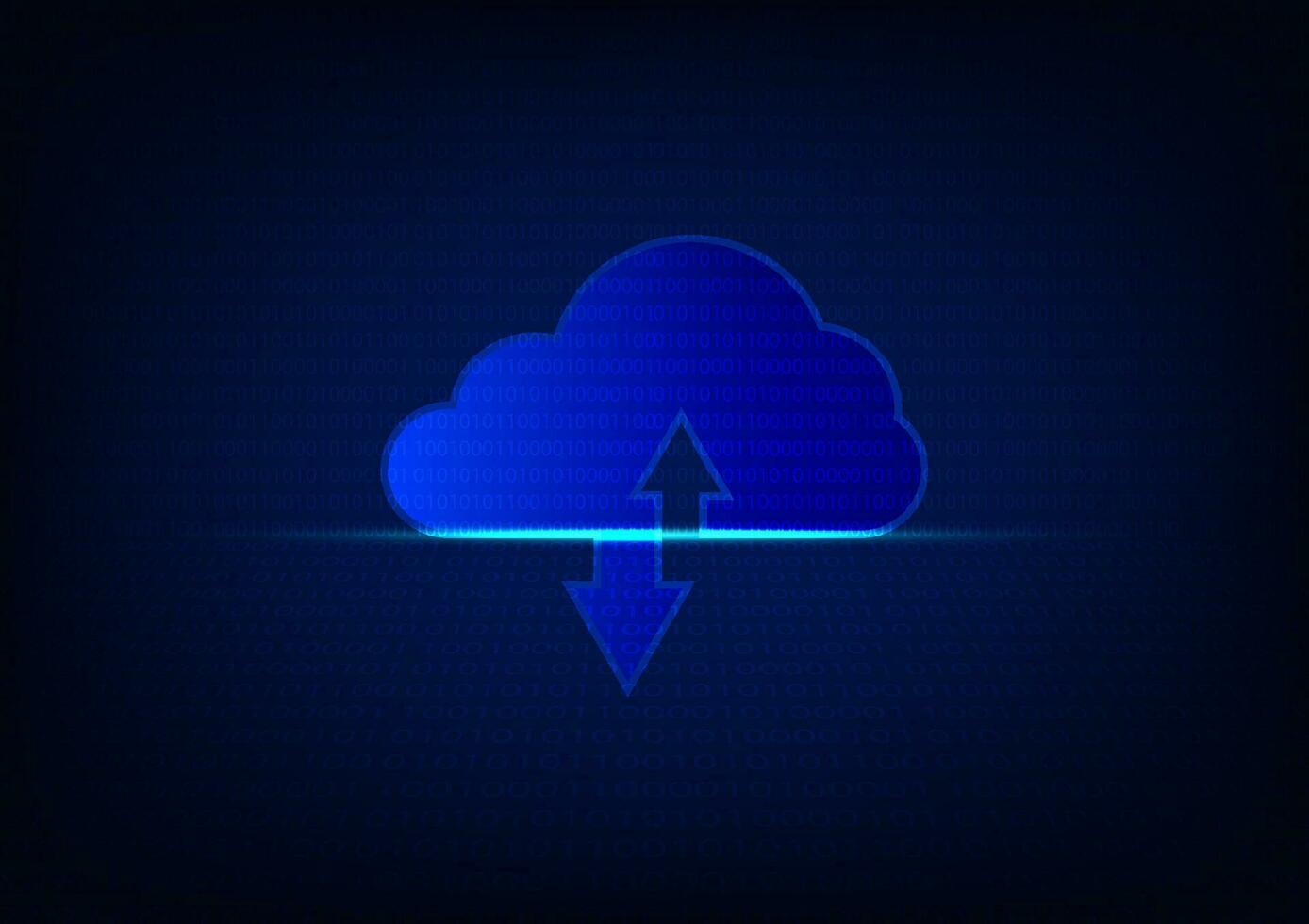The image is a close-up screenshot of an icon resembling a cloud with upload and download functions. The background is a gradient of midnight blue to lighter blue, highlighting the central cloud motif. The cloud itself is bright royal blue with two arrows: a dark blue arrow pointing up from the bottom and a light blue arrow pointing down underneath the cloud. The icon appears pixelated, suggesting it has been enlarged. A horizontal line runs through the image, gradually transitioning from dark to turquoise before fading back to dark, indicating the button's selection or hover state. The backdrop is adorned with indecipherable binary text, adding a digital touch to the composition.